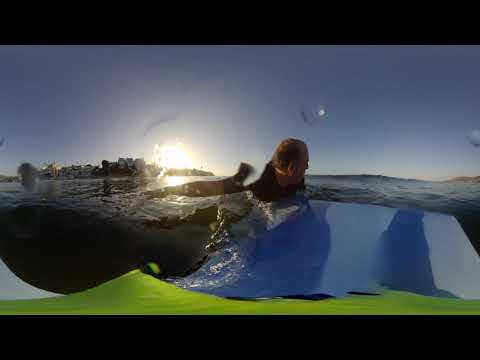A man dressed in dark-colored clothing is partially submerged in calm, dark blue water, with only his head visible. He seems to be paddling towards or on a flat object that is adorned with light blue, dark blue, and white stripes, possibly a surfboard or raft. The serene water presents splashes around him, adding dynamic movement to the scene. In the background, a panoramic view reveals a cityscape and obscure rock or building structures under a stunning sunset. The sun, appearing white against the backdrop of a fading blue sky, casts a blue hue over distant mountain ranges. Flanked by a couple of black lines at the top and bottom edges, the overall image is tranquil yet lively.